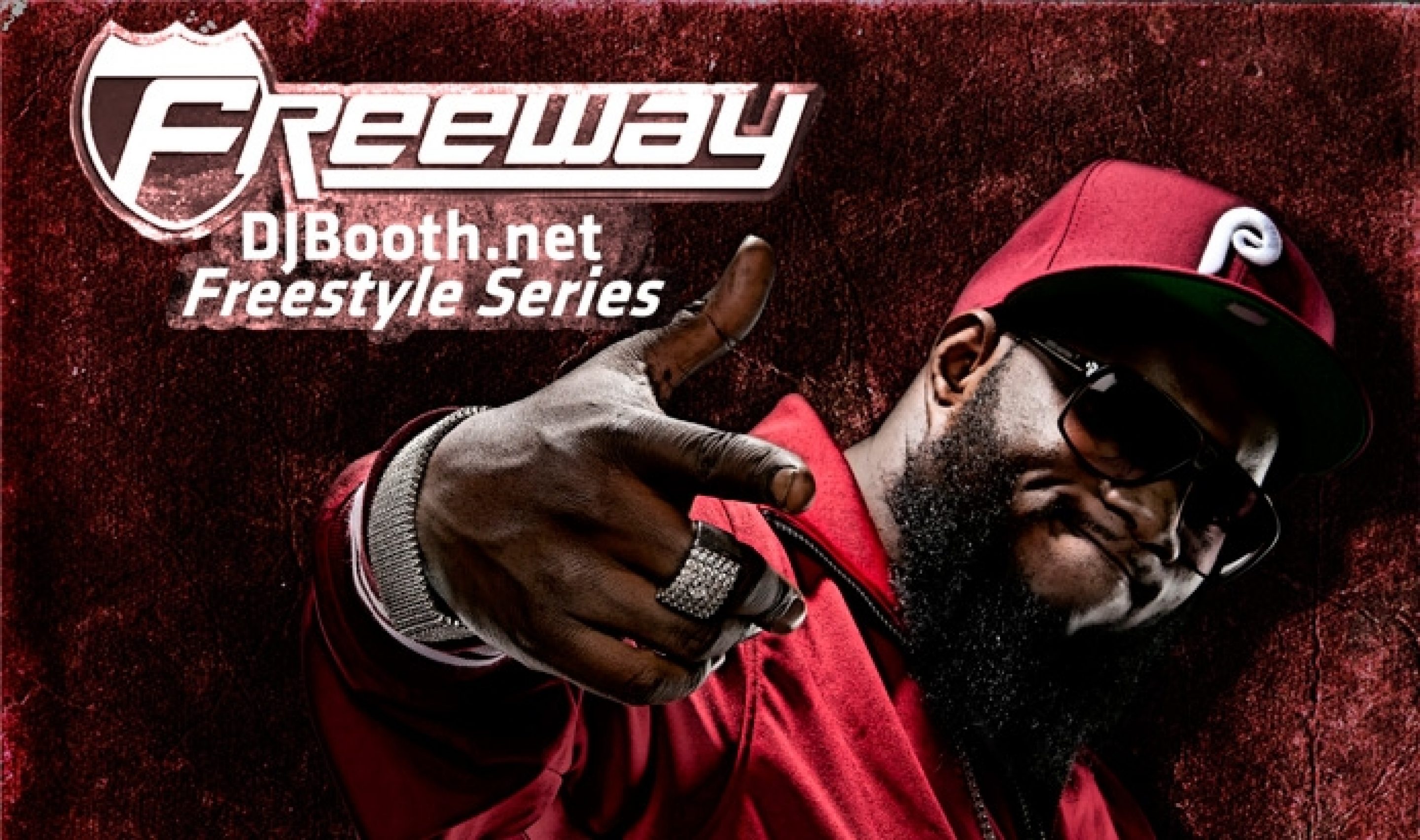The advertisement banner highlights an African American artist poised dramatically against a dark, red textured background that resembles brick or concrete. Dominating the visual, the artist extends his hand towards the viewers, adorned with a large diamond ring on his middle finger and a flashy jeweled watch or bracelet on his wrist. His stern expression, accented by a black beard and pursed lips, is partly concealed by gradient brown sunglasses. He wears a red Phillies baseball cap and an unzipped red hoodie, adding to his striking appearance. Positioned in the top left corner is a stylized Freeway logo, resembling an interstate sign with an 'F', and the words "Freeway DJBooth.net Freestyle Series" are clearly displayed in white text, marking the advertisement's primary focus.